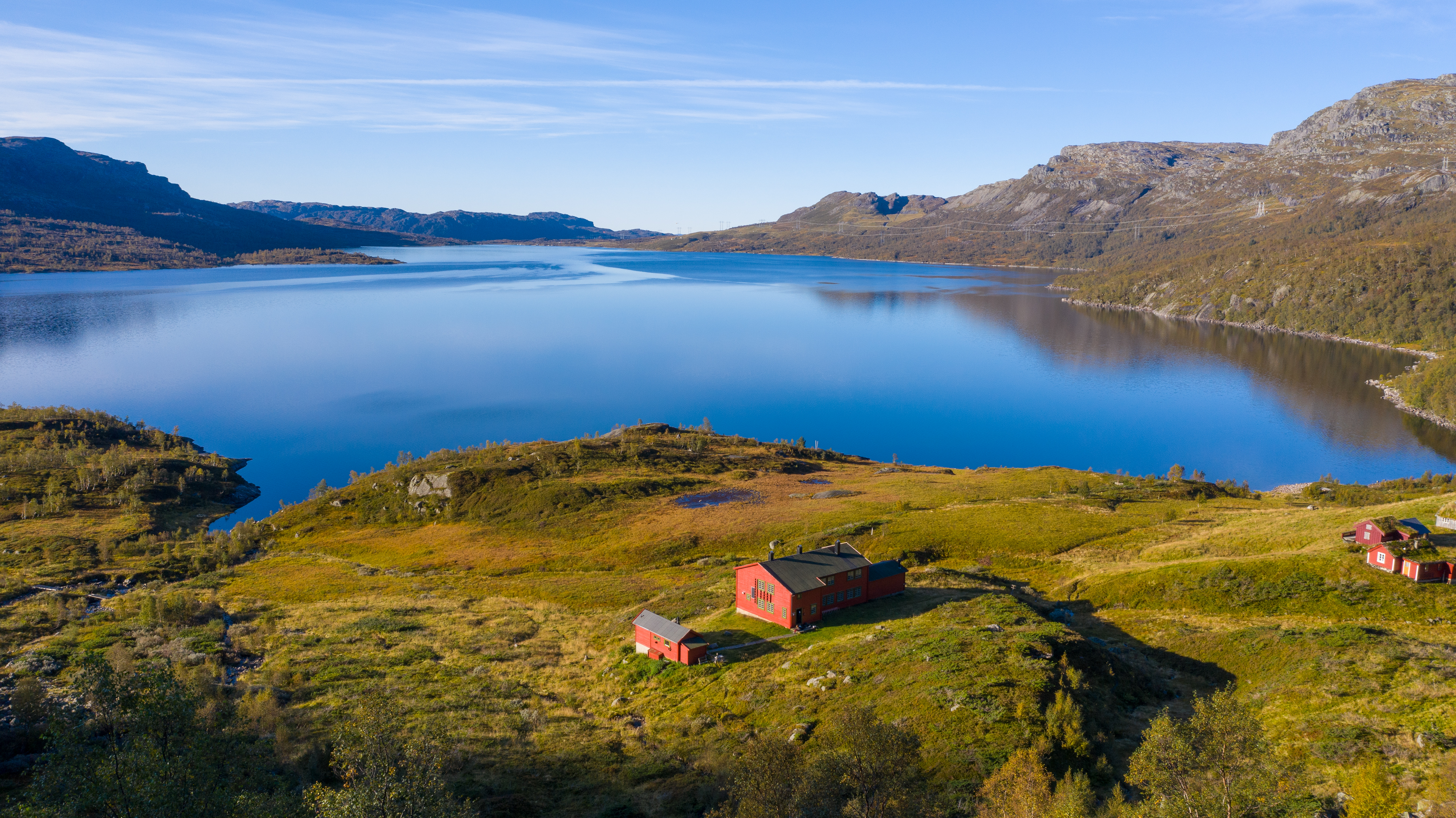This photograph captures a serene lake nestled within a mountainous landscape. Dominating the bottom half of the image are lush green shores with scattered shrubs and small trees, leading to the lake's edge. The calm, glassy surface of the lake reflects the vibrant blue sky adorned with wispy clouds, creating a mirror-like effect. Central to this bucolic scene is a prominent red building with a flat black roof and a few chimneys, likely serving as either a barn or a large house. Adjacent to the main building on the left is a slightly smaller red structure, while the right side of the photograph features additional smaller red buildings with white trim. These structures cast long shadows over the vivid green grass, indicative of either early morning or late afternoon sunlight, which streams into the frame from the left. The background reveals rocky, moderate-height mountain faces, adding a majestic yet calming backdrop to this picturesque tableau.